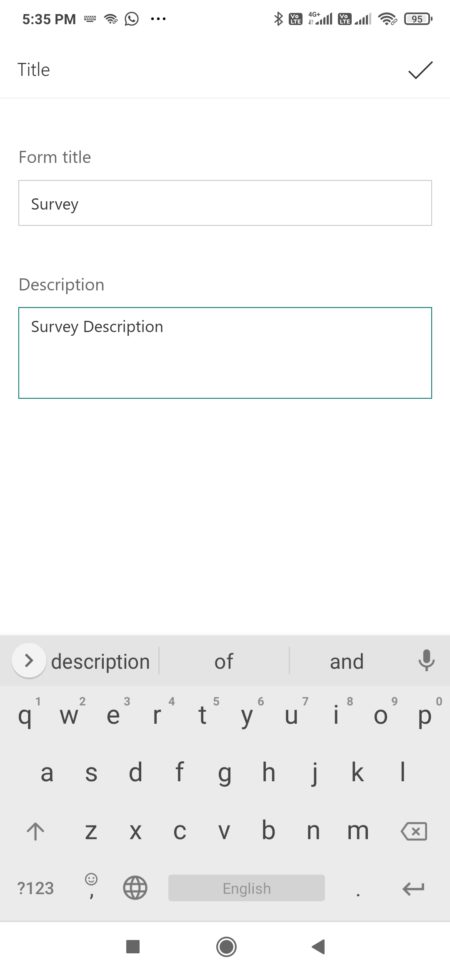A detailed screenshot of a cell phone interface:

The image features a white background with text displayed in either black or grey. At the top left corner, the time "5:35 PM" is shown in bold black font. Adjacent to the time, there's a small keyboard icon. Moving further right, a series of status icons include: a Wi-Fi signal indicator, a text bubble with a phone receiver, and three horizontal grey dots.

On the right-hand side of the status bar, several grey icons are present, including a Bluetooth signal. There's also a small black square with unreadable white text. Positioned above five bars representing Wi-Fi strength, the "4G" label is visible. Another grey square with the text "LTE" shows four out of five bars, accompanied by a Wi-Fi signal indicator. Lastly, a grey battery icon displays "95" in grey lettering inside it.

Below the status bar on the left side of the screen, there's a title. On the far right, a grey checkpoint or a check mark is visible. Beneath this, another grey title is labeled “Form Title” on the left, and a grey-outlined rectangle contains the word "Survey" in black text. Below that, the word "Description" appears in black text, followed by a blue-outlined rectangle with bold black lettering stating "Survey Description."

At the bottom of the screen, a grey background keyboard is visible, typical of the Google keyboard layout in QWERTY fashion. At the very bottom, there are three icons: a grey-black square on the left, a red-black circle in the center, and a black left-facing arrow on the far right.